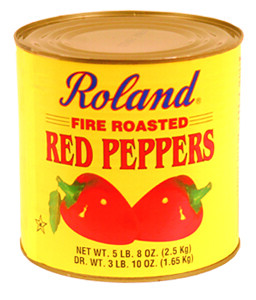The image features a gold tin can against a white background. The can is adorned with a yellow label, prominently positioned in the center. At the top center of the label, "Roland" is written in blue with a red outline. Directly below this, the text reads "Fire Roasted Red Peppers" in bold red letters. The bottom section of the label displays an illustration of red peppers, arranged with their tips pointing outward and stems oriented towards both the right and left sides. Additional information is provided beneath the illustration: "Net Wt. 5 lb. 8 oz (2.5 kg)," followed by "Dr. Wt. 3 lb. 10 oz (1.65 kg)" indicating the drained weight of the contents. The top and bottom edges of the can each feature a subtle gold ring, framing the label neatly.